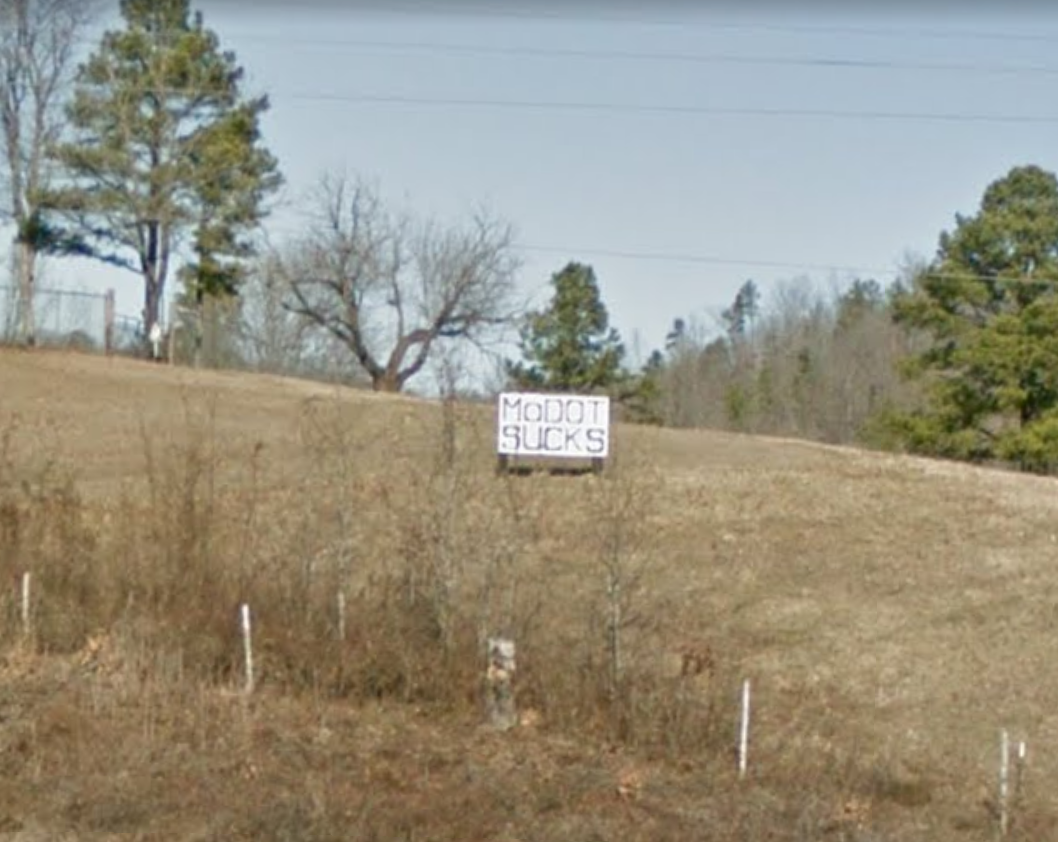The photograph, taken outdoors in low resolution, captures a barren scrubland field dominated by yellowish, dead grass or straw. The foreground features barren hedgerows curving slightly from the left bottom third to the bottom right corner, composed primarily of brown twigs and some thin trunks with white bark. Central to the image is a white homemade sign with black lettering, reading "MoDOT SUCKS." The backdrop includes a mix of dead and green-leaved trees, with green foliage more noticeable and taller trees scattered across the background. Additionally, telephone or power lines stretch left to right across the upper third of the photograph. We can also see sparse fencing elements, marked by white posts at the bottom front of the image, hinting at a barely visible fence line. The sky is blue, offering a clear atmosphere over the desolate landscape.